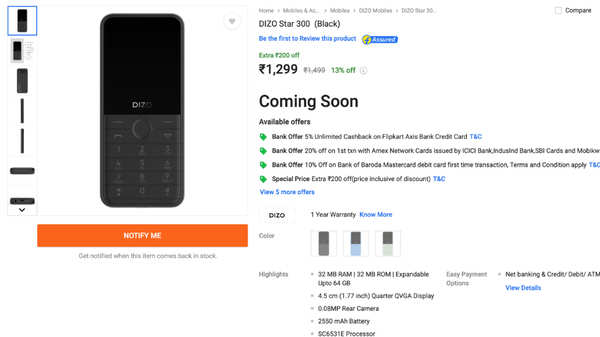This image is taken from a website where a person is considering purchasing a device, presumably a cell phone. The device is identified as the "Dizzostar 300 Black." Though the full name isn't wholly clear on the screen, it prominently displays the partial text "DIZ" in faint letters. This device, with its sleek black design, occupies the main segment of the picture on the left.

To the left side of the screen, there are clickable areas that provide additional information and more photos of the device. At the bottom of the image, an orange box with white text contains the option "Notify Me," which prompts users to get notifications when the item is back in stock.

The top of the image displays the price as $1,299, though the currency symbol isn't identified. Additional information includes a one-year warranty, a "coming soon" status, and available offers prominently mentioned.